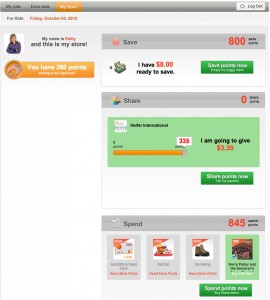This is a small, slightly blurry image of a vertically rectangular webpage. At the top of the page, there's a thin gray ribbon with black text on the left that seems to start with "my," followed by some additional text that is too tiny to read. On the far right of this ribbon, there is a white button with black text that reads "Log out."

Below this ribbon, there is another horizontal section on a gray background. On the left side of this section, there is light gray text saying "For Kids," while to the right, there is some red text that is also too tiny to read.

Beneath this section, on the left side, there is a square profile picture with a white background. The profile image features a woman wearing a dark gray shirt, with her arms folded in front of her. She has light brown hair. To the right of this image, there is black text that reads "My name is Emily and this is my store!" with the name "Emily" highlighted in red.

Below this message, there is an orange button that says, "You have 200 points waiting to be registered." To the right of this profile and button area, there appears to be a large amount of additional content, though details of this content are not specified.